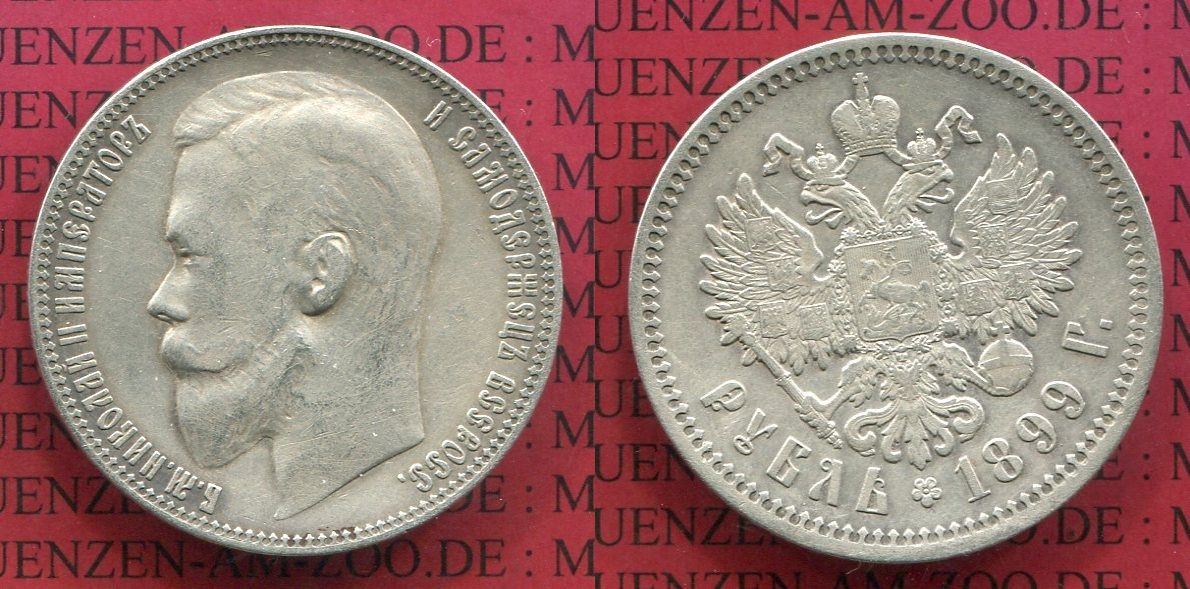This image showcases both sides of a silver coin, set against a red background with indistinct, foreign writing, possibly ending in ".E.D.E". On the left side, the obverse features a detailed left-side profile of a man with a prominent mustache, short hair, and a sharp nose. The edge is adorned with unreadable Cyrillic script. On the right, the reverse side displays a double-headed eagle with a crown. The eagle clutches a key in one claw and a globe topped with a cross in the other. At the center of the eagle is a shield depicting a man on horseback. Surrounding the imagery are additional foreign inscriptions, including the year "1899" at the bottom.